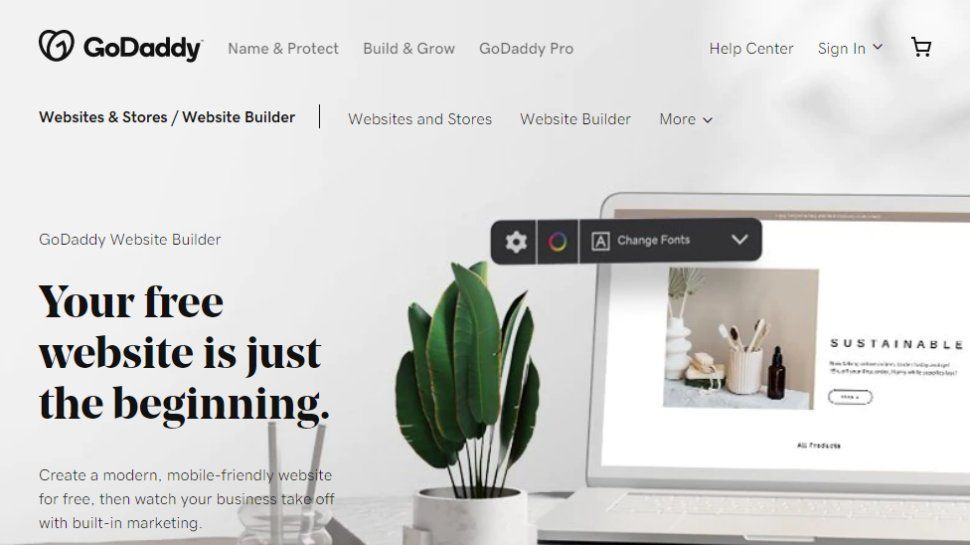The image is an advertisement for GoDaddy's website services. At the top, the GoDaddy logo is prominently displayed alongside navigation options: "Name and Product," "Build and Grow," "GoDaddy Pro," "Help Center," "Sign In," and "Cart." Below this navigation bar is a menu with sections labeled "Websites and Stores," "Website Builder," and a "More" option indicated by a downward arrow.

The central focus of the advertisement is a large, bold headline stating, "Your free website is just the beginning." This text is the largest on the page, emphasizing the initial free offering. To the right of this headline, there's an image of a white planter with a thriving plant, featuring dark, healthy green leaves.

On the left side of the page, a subheadline reads, "Create a modern, mobile-friendly website for free, and watch your business take off with built-in marketing." This highlights the convenience and marketing tools included with their website builder.

To the right, a visual showcases a laptop next to various artist tools. These tools include brushes in a container and what appears to be items related to hairstyling or nail care, indicating the versatile applications of their services. Below this, the word "Sustainable" is partially visible, though the remaining text is too small to read clearly.

Overall, the ad emphasizes the ease of creating a visually appealing and mobile-friendly website with GoDaddy, complete with marketing tools to help businesses grow.